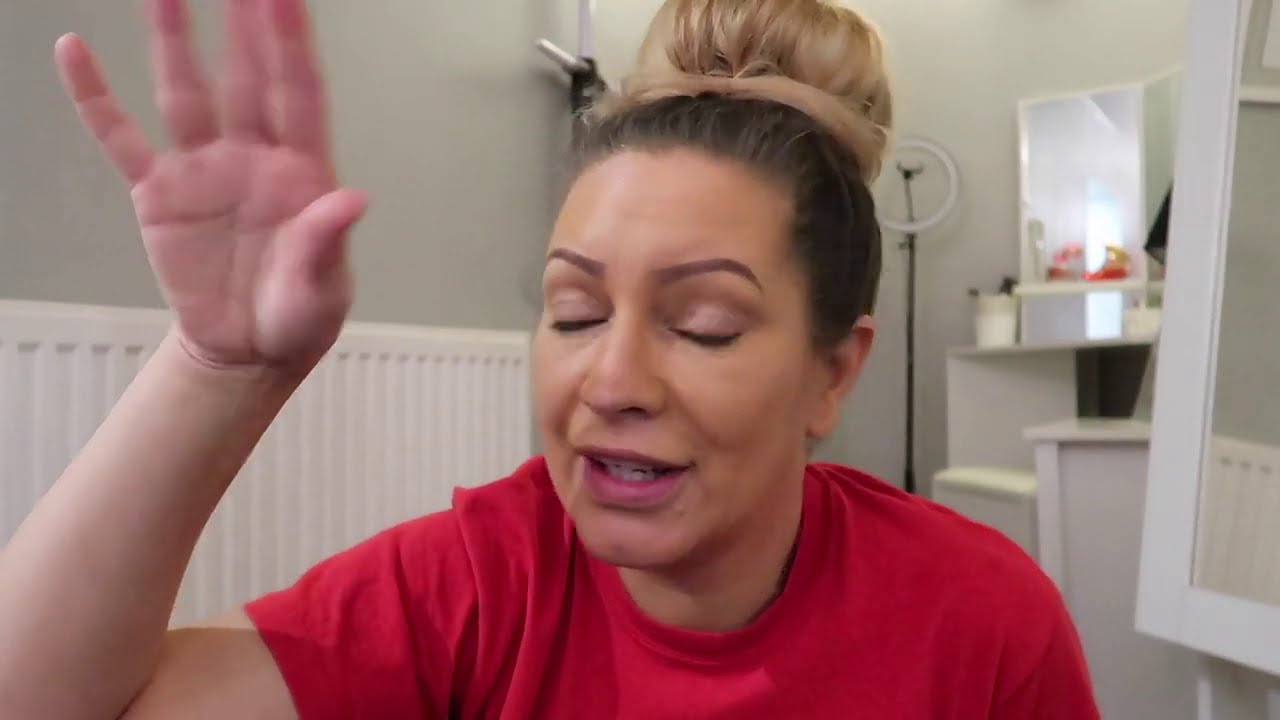In the photograph, a woman with brunette hair tied up in a bun, with light brown to dark blonde extensions or a wig on top, is captured in the midst of speaking. Her right arm is raised to about eye level, her hand gesturing as if to emphasize her words. She has pink lipstick on her slightly open lips, revealing her teeth, and her eyes are closed. Her sharply defined eyebrows, almost appearing hand-drawn, give her a striking look. She is wearing a red t-shirt and appears to be slightly tanned. The setting suggests she is in a bathroom, with tan walls and a white lower half indicating some form of a shelf behind her. To her right, the presence of a mirror and a ring light can be seen, along with cabinets against light green walls with a textured white lower section. The overall scene gives off the impression she is humorously discussing something, potentially the blonde additions to her hair.